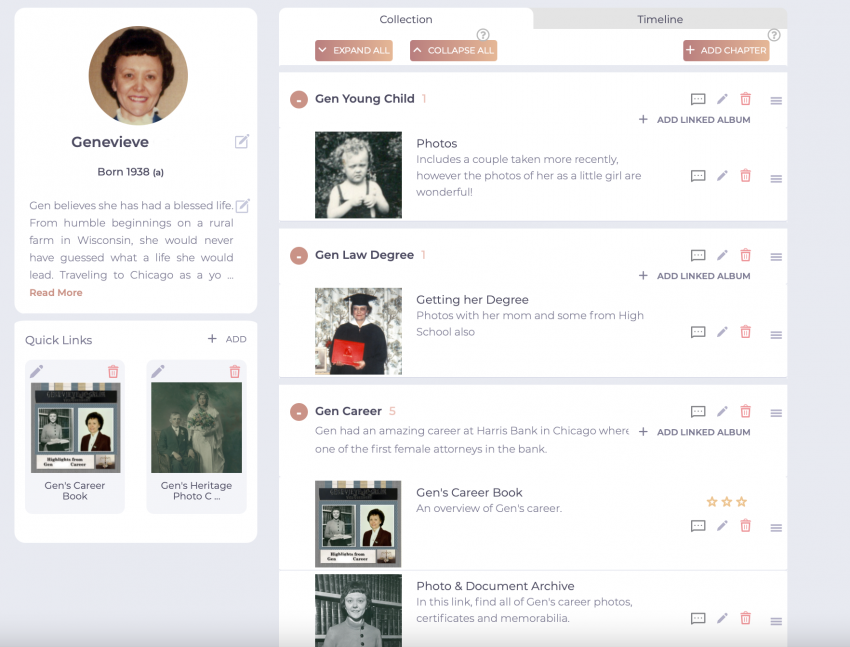This image depicts a screenshot from either a biography page on a website or a social media profile, chronicling the life of a woman named Genevieve. 

On the left side of the page, two white boxes present biographical details about Genevieve. The first box is topped with a portrait of an older woman, seemingly taken in the 1960s or 1970s. Below the picture, in gray text, the name "Genevieve" is displayed, followed by "born 1938 (A)," implying an estimated birth year. Beneath this, a brief biography about Genevieve is provided, succeeded by a red link labeled "Read More," inviting users to delve deeper into her life story.

At the lower left, another white box features the text "Quick Links" in gray, offering shortcuts to "Gen's Career Book" and "Gen's Heritage Photo Collection."

The center of the page is dominated by a large column filled with multiple white boxes, each containing links to various aspects of Genevieve's life. These include headings like "Gen Young Child," "Gen Law Degree," and "Gen Career," providing insights into her personal and professional milestones. The section also includes several vintage photographs, some in black and white and others with minimal color. These images capture moments from her life, such as her time with her mother and son during high school, an overview of her career, and details about her certificates and memorabilia.